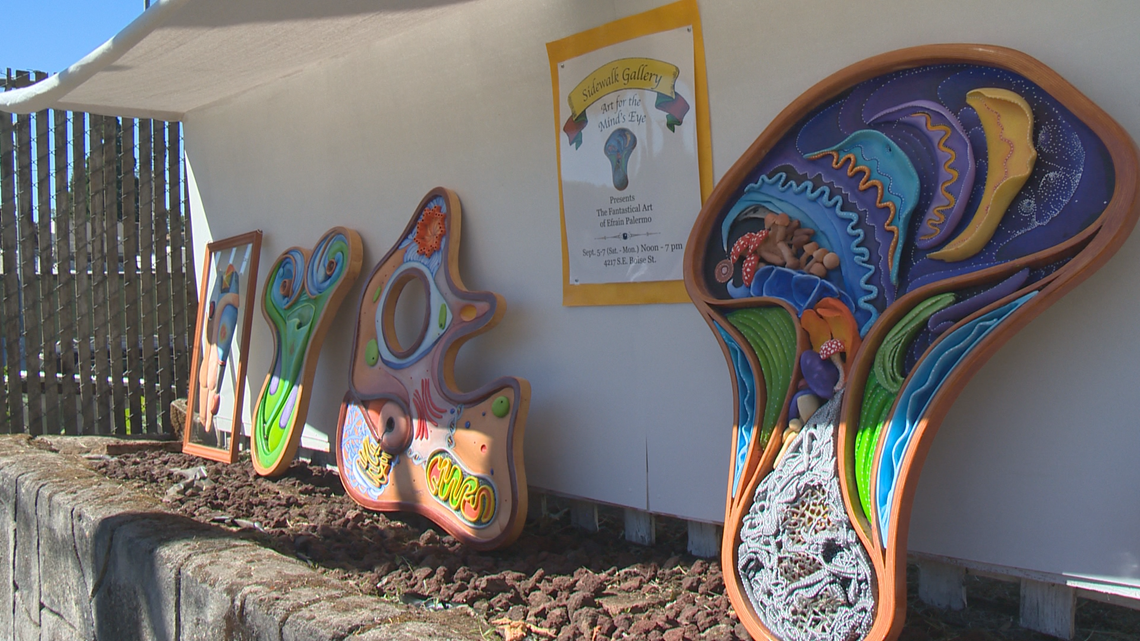The image depicts the exterior of a gallery, identified as the Self-Folk Gallery, indicated by an orange poster on a white makeshift wall. Below the gallery sign, there are some pieces of writing that aren't legible. The scene is set against a brick wall adorned with a planter featuring gray and red stones. Several abstract art pieces are leaning against this wall, showcasing a variety of shapes and vibrant colors.

On the far right, there's a mushroom-shaped sculpture with intricate squiggles and a mix of greens, blues, purples, and whites. Next to it is an oddly-shaped piece with a hole in the center, followed by another art piece resembling a heart with an elongated bottom, painted in green and blue with what appear to be two eyes. Further to the left, there's a framed piece with an abstract design hanging within it, surrounded by hues of blues, greens, purples, peaches, and reds.

These sculptures, possibly made from clay or materials reminiscent of Play-Doh, are colorful and playful, giving off a childlike charm. They are placed on a stone shelf-like structure, which adds a rustic touch to the gallery's exterior. In the background, a fence is visible along with the blue sky above, completing the setting for this eclectic outdoor display of abstract art.